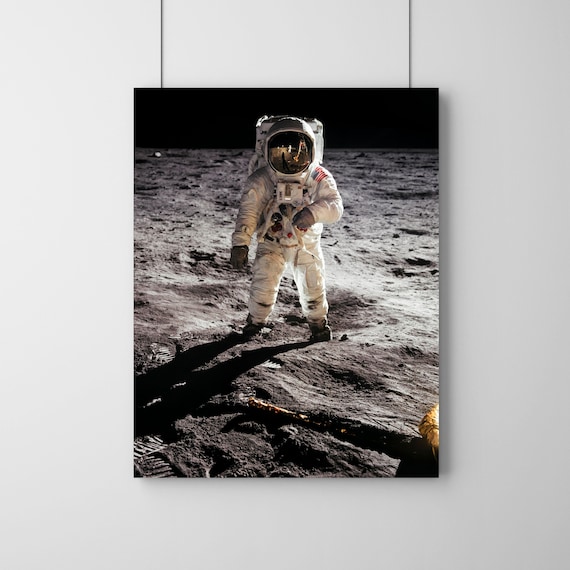The image depicts a captivating and iconic scene of an astronaut taking monumental steps on the moon's rocky and sandy surface. The astronaut, dressed in a pristine white spacesuit adorned with an American flag, is captured mid-stride, walking towards a partially visible golden object in the lower right corner and leaving behind discernible tire treads on the bottom left. His shiny, reflective helmet mirrors the high-definition environment, casting shadows from the light source on the right side of the photo. This historic image is printed possibly on canvas and mounted prominently against a light-colored wall, described variably as white, beige light olive, and very light gray. The photograph is suspended by two black ropes or cords attached to the top corners, giving it an unframed, yet strikingly attention-grabbing display.